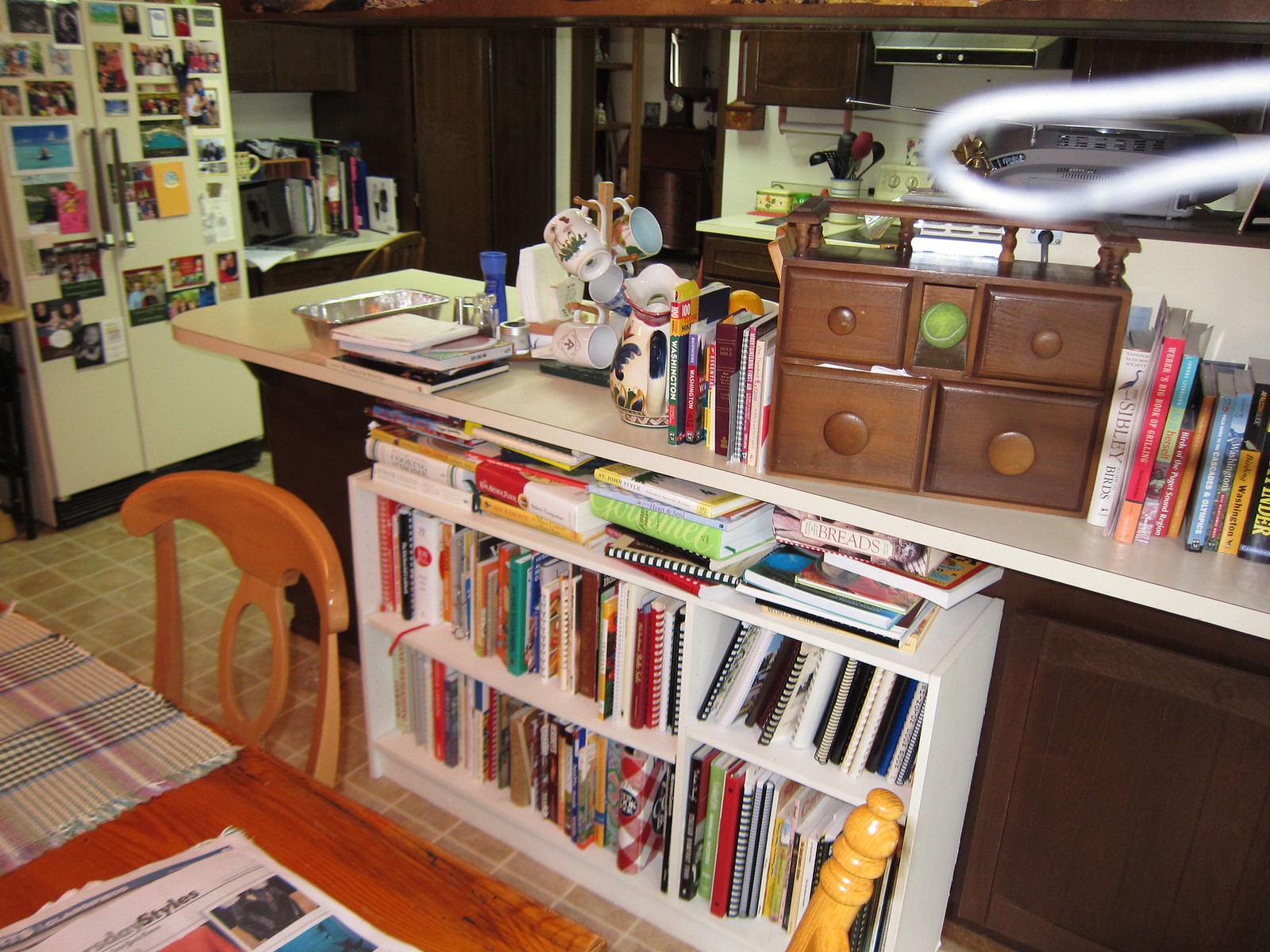In this vibrant and eclectic kitchen-dining room, a myriad of colors and objects catch the eye, creating a warm and lived-in atmosphere. Dominating the foreground is a large white bookshelf nestled under the kitchen island, filled with an array of books in red, teal, orange, white, yellow, and more. Above this bookshelf stands a compact wooden storage unit with four drawers, curiously adorned with a tennis ball in its center. Encompassing the wooden drawers are additional stacks of books, extending left and right.

To the left of the storage unit, a quaint mug tree holds a collection of mugs, accompanied by a glass and a porcelain jar for pouring drinks. Further left, an off-white, nearly beige fridge is adorned with a myriad of magnets and personal photos, adding a touch of nostalgia and personality to the scene.

Behind the wooden compartment and bookshelf, the kitchen area gradually comes into focus, revealing an oven and a stove. An adjoining walkway on the left suggests access to another part of the home. In front of the bookcase, a wooden table and matching chair stand ready for use, with a newspaper laid out across the table's surface, hinting at a leisurely morning or evening read. Multiple tablecloths add a cozy touch to the setting. In the background, even more books sit beside the fridge, continuing the theme of a home where reading and culinary arts joyfully intersect.